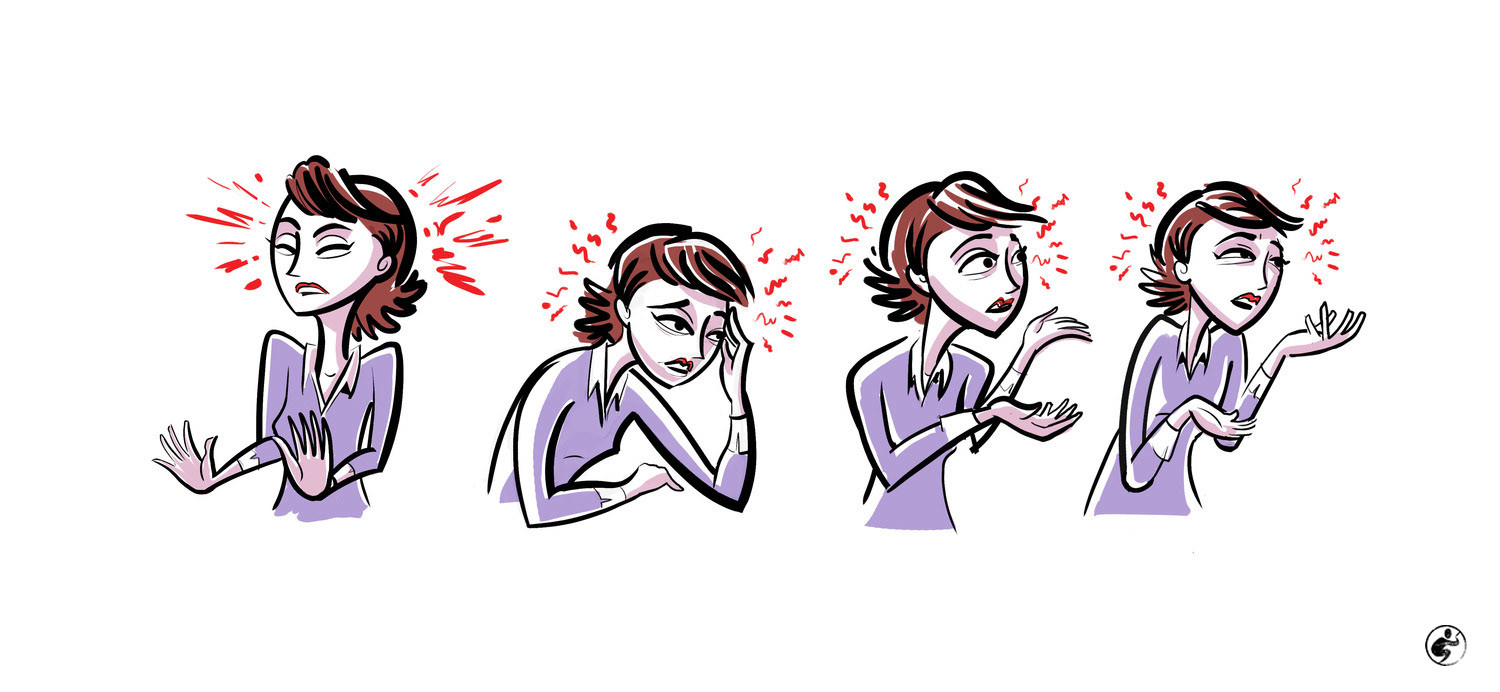The image is a detailed cartoon collage depicting a woman experiencing various stages of a headache. The background is white and the collage consists of four pictures aligned side by side. The woman has short brown hair and is dressed in a purple blouse. 

In the first picture on the left, she stands with her hands extended out to her sides, palms open, and her eyes closed. Red lines emanate from her head, indicating the onset of a headache. In the second picture, she is hunched over with one hand resting on a desk and the other on her forehead, suggesting an intensifying headache, with the same red lines emphasizing her pain. 

The third image shows her in a distressed state, making circular motions with her hands, looking disheveled and flustered, again accompanied by the red squiggles. In the final pane, she appears even more distressed, with eyes almost completely closed and hands closer to her body, encapsulating the severe discomfort of the headache. The overall composition vividly captures the progression of her headache through varying body language and expressions.